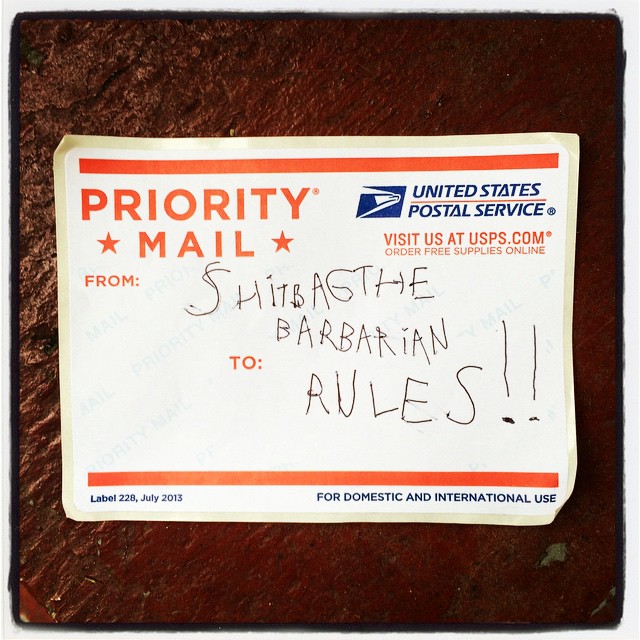The image is that of a United States Postal Service Priority Mail sticker affixed on a rough, weathered, dark brown wooden surface. The sticker is rectangular and oriented horizontally, with red stripes at the top and bottom. In the upper left corner, it reads "Priority Mail" flanked by red stars, while the upper right corner states "United States Postal Service" followed by "Visit us at USPS.com. Order free supplies online." Below this, there is a section with “From” and “To” fields. In the "From" field, handwritten in what resembles a childish scrawl, it reads "Shitbag the Barbarian." The "To" field contains the words "Rules!!" in a similar handwriting style. The bottom left corner of the sticker is marked “Label 228, July 2013,” and the bottom right notes "For domestic and international use."